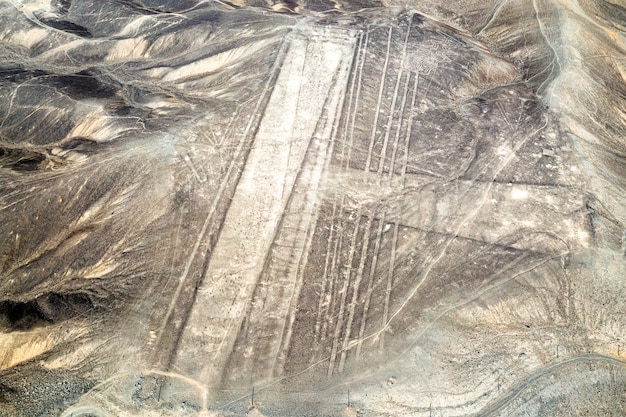The photograph is an aerial shot of a barren, mountainous landscape that resembles either a snow-covered region or a desert terrain. Dominating the left side of the image are long, wispy strands that look remarkably like clumped, wet hair, particularly visible in the top left corner. Moving towards the center, the terrain features various hills and a notable star-shaped formation with a circled center and eight radiating lines. The starkly detailed textures and scratches on the surface resemble the fine patterns and etchings of marble stones, exhibiting a range of colors from white and gray to tan and brownish-gray. 

In the bottom right corner, there is a clearly visible road or airstrip that appears to be gravelly and winding, surrounded by ridges that slope downward. Additionally, the photograph portrays intricate lines and markings, seen as either natural formations or man-made roads and pathways. Some of these lines have a muddy, dirty tarp-like appearance, enhancing the imagery of the landscape being worked on or excavated.

The image’s overall impression is both surreal and topographical, with elements identifiable as tree trunk roots or timber entwined within the landscape, reinforcing the resemblance to either a marbled painting or a black and white photograph of a snow-clad expanse.